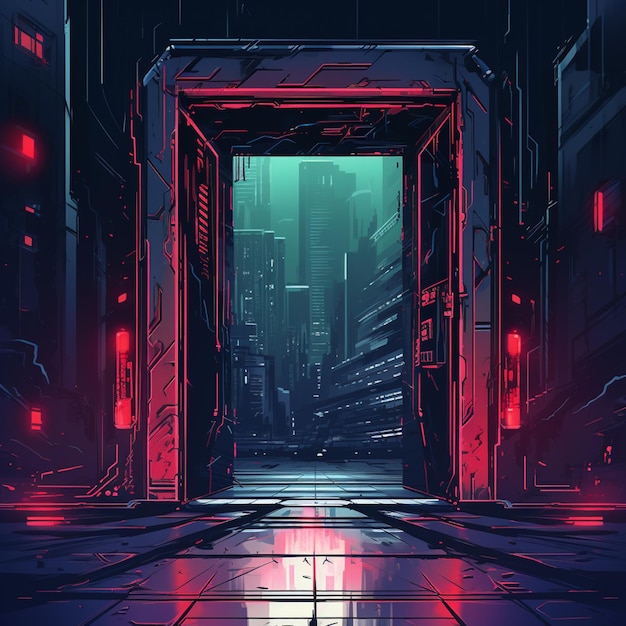In the image, you find yourself inside a large, modernistic, and futuristic metal room. The walls are covered in a combination of dark blue and purple hues, illuminated by red lights that cast intriguing reflections, creating shades of blue and pink on the shiny, mirrored tile floor. The room is filled with metal piping and various types of machinery, suggesting a high-tech environment. At one end of the room, there is a large, thick, rectangular arch doorway, which appears to function possibly as an elevator or control room, with intricate controls for managing doors. Through this archway, you can see a sprawling cityscape outside, filled with buildings of varying heights, distinguished by their numerous windows and lights. The exterior scene is dark and somewhat black-and-gray, with tall, slender structures juxtaposed against massive, looming buildings, all contributing to the distinctly futuristic and cinematic atmosphere.